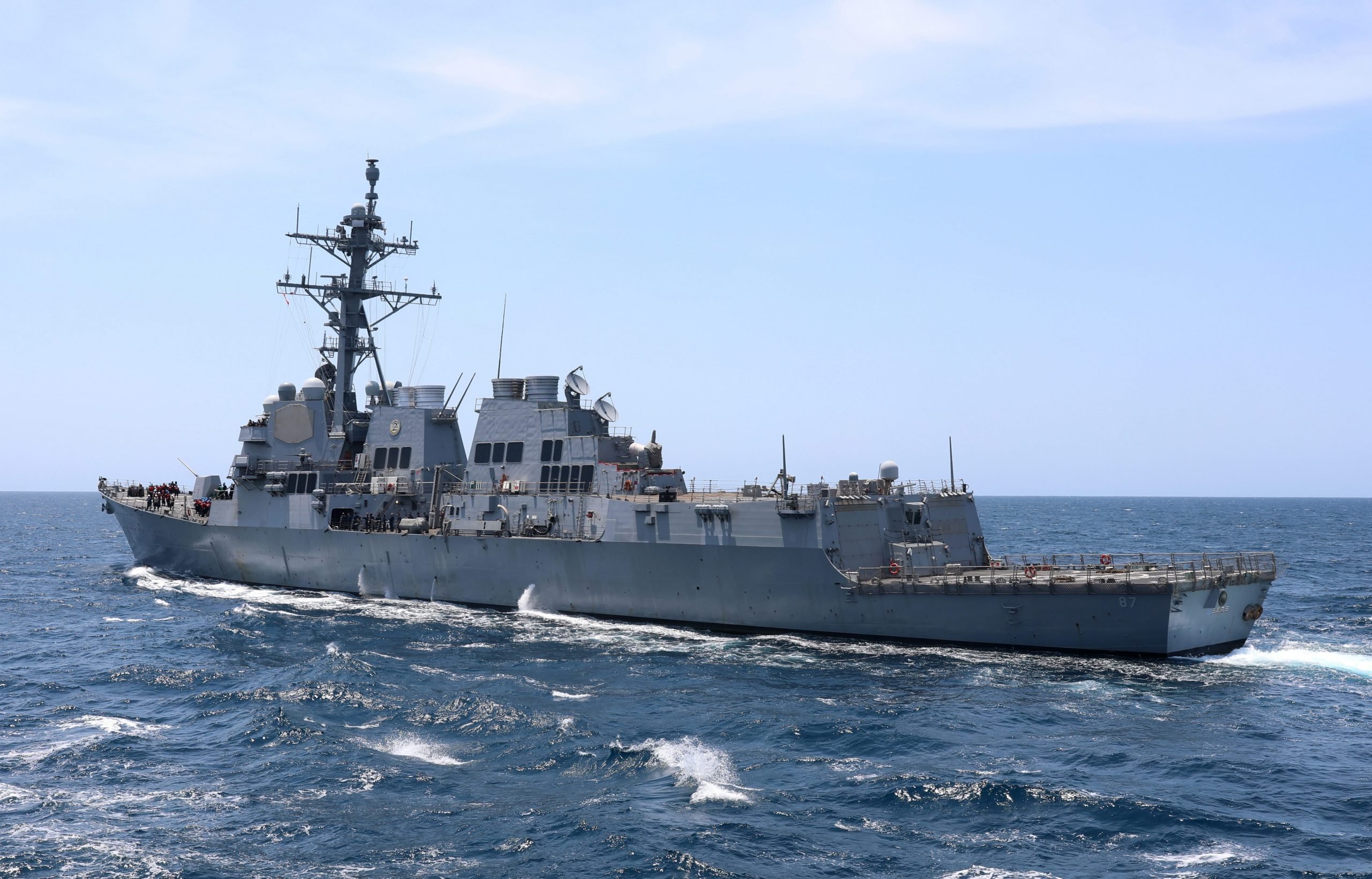The image depicts a large, high-tech naval battleship, identified by the white number "87" on its bottom right side. The vessel, a gray-silver color with varying shades of blue, beige, and gray, spans a significant length and features distinct structural elements: a flat stern, a central section with towers and various satellite dishes, antennas, radar spires, and related equipment, as well as a flat bow with high poles. The middle section also displays the number "2." The ship is equipped with many windows, lifeboats along the side, and lifeguard equipment on the guide rails. At the very back, there appears to be a landing platform, likely for helicopters. The image captures a clear day with a blue sky scattered with a few white clouds, and deep blue ocean waters dotted with white wave crests. The relatively calm yet slightly turbulent sea accentuates the immense scale of the ship, further highlighted by the small figures of people visible on board.